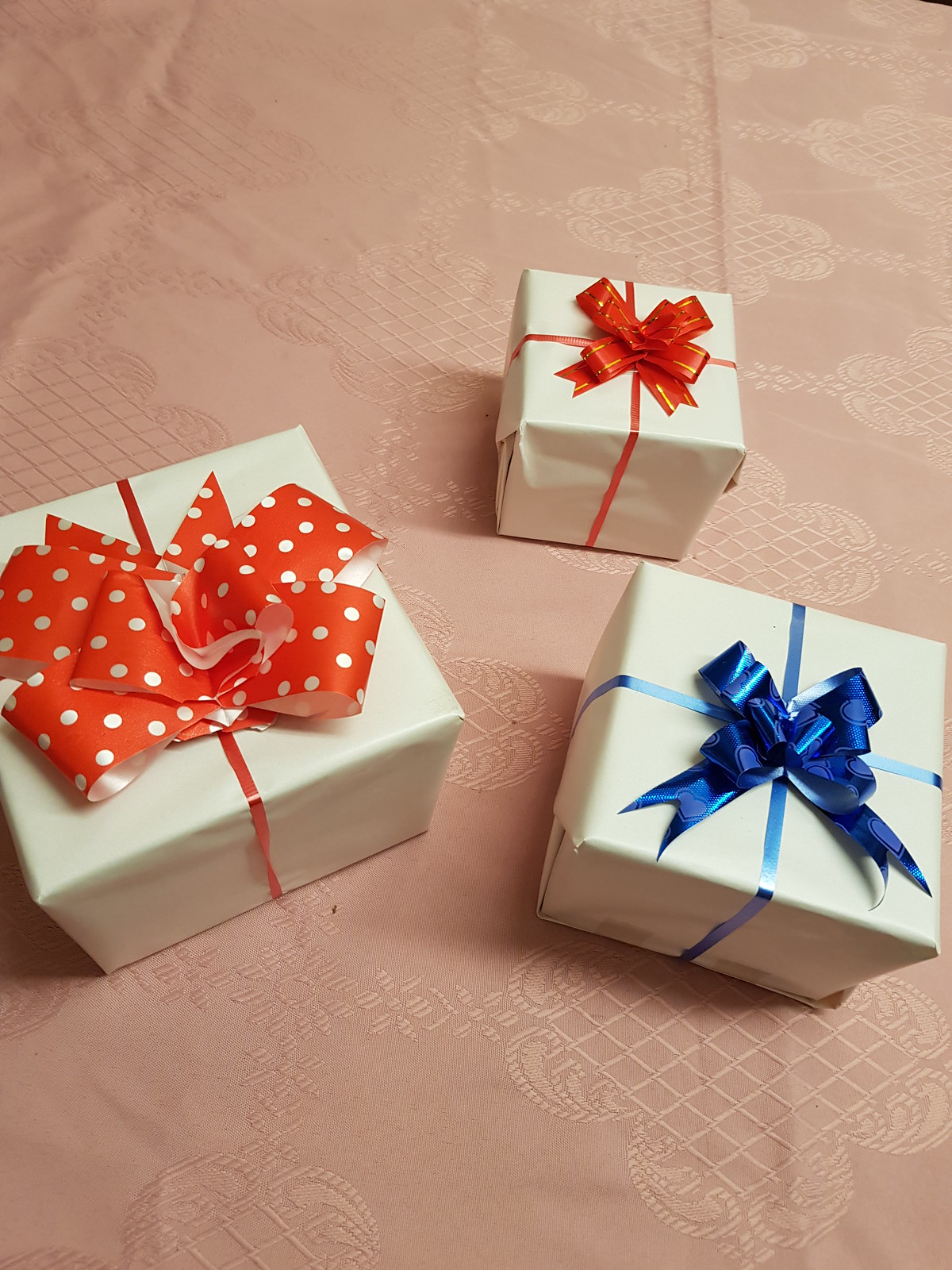This photograph captures three intricately wrapped presents arranged on a peach-colored, intricately embroidered cloth that features a subtle flower-like square grid pattern. On the left side of the image, there is a present wrapped in white paper, adorned with a large red bow with white polka dots and a simple red strap. Beside it, there is a smaller package, also in white wrapping paper, distinguished by its plain red bow and two crisscrossing red straps. In front of this smaller package is a slightly larger box wrapped in the same white paper, featuring a metallic blue bow with light blue hearts and two crisscrossing metallic blue straps. The detailed bow trims and careful ribbon work accentuate the festive and meticulous presentation of these gifts.